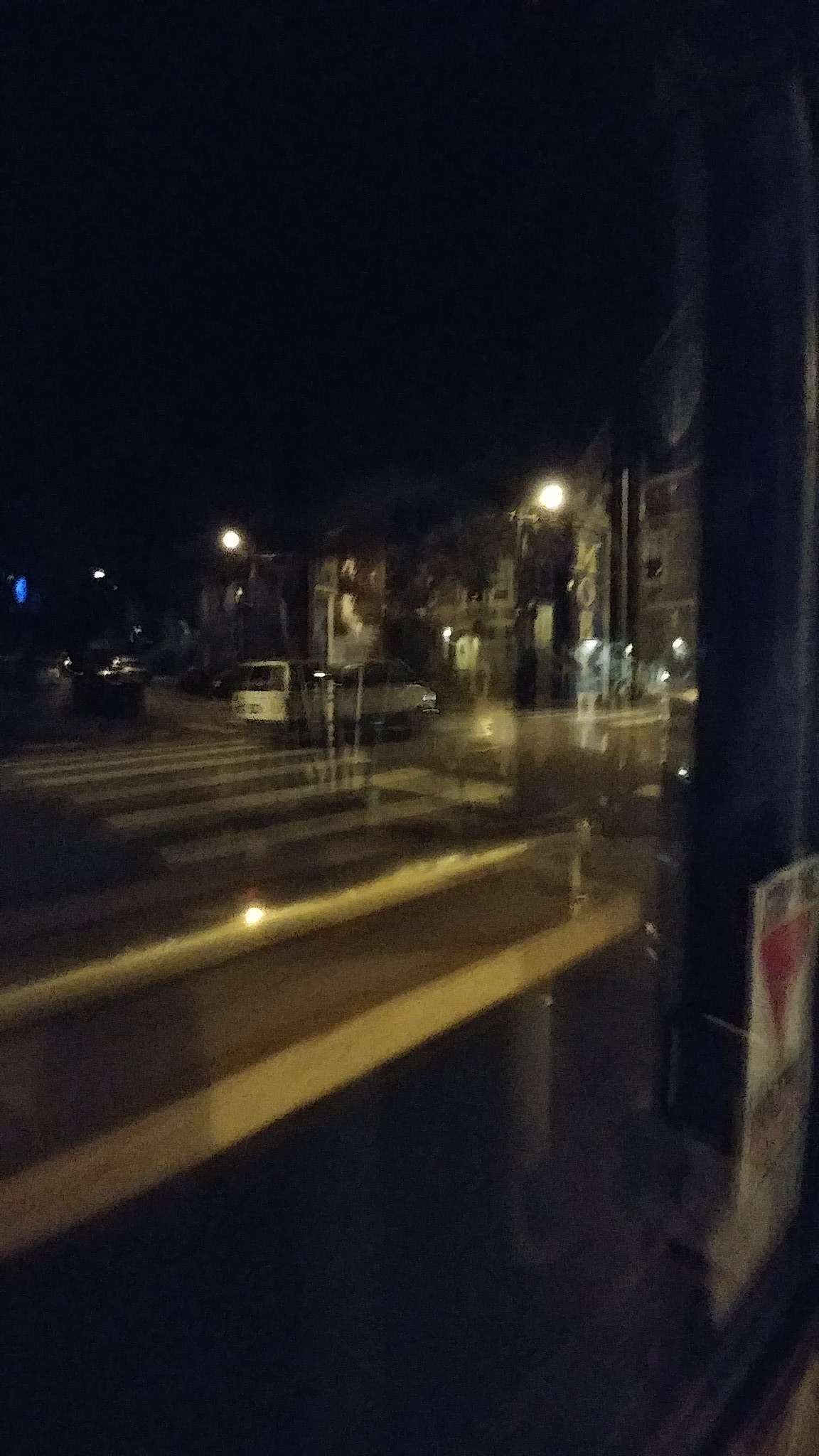This blurry nighttime photograph captures a city street scene through a reflective window. The dark sky and indistinct outlines of buildings set a moody atmosphere, while the faint, scattered streetlights provide modest illumination. The presence of a crosswalk suggests pedestrian activity, although there are no people visible. The image also includes several cars in motion, further contributing to the dynamic urban setting. The photograph is taller than it is wide, emphasizing the vertical stretch of the scene. Despite the lack of clear details, the image evokes a sense of nocturnal urban life.